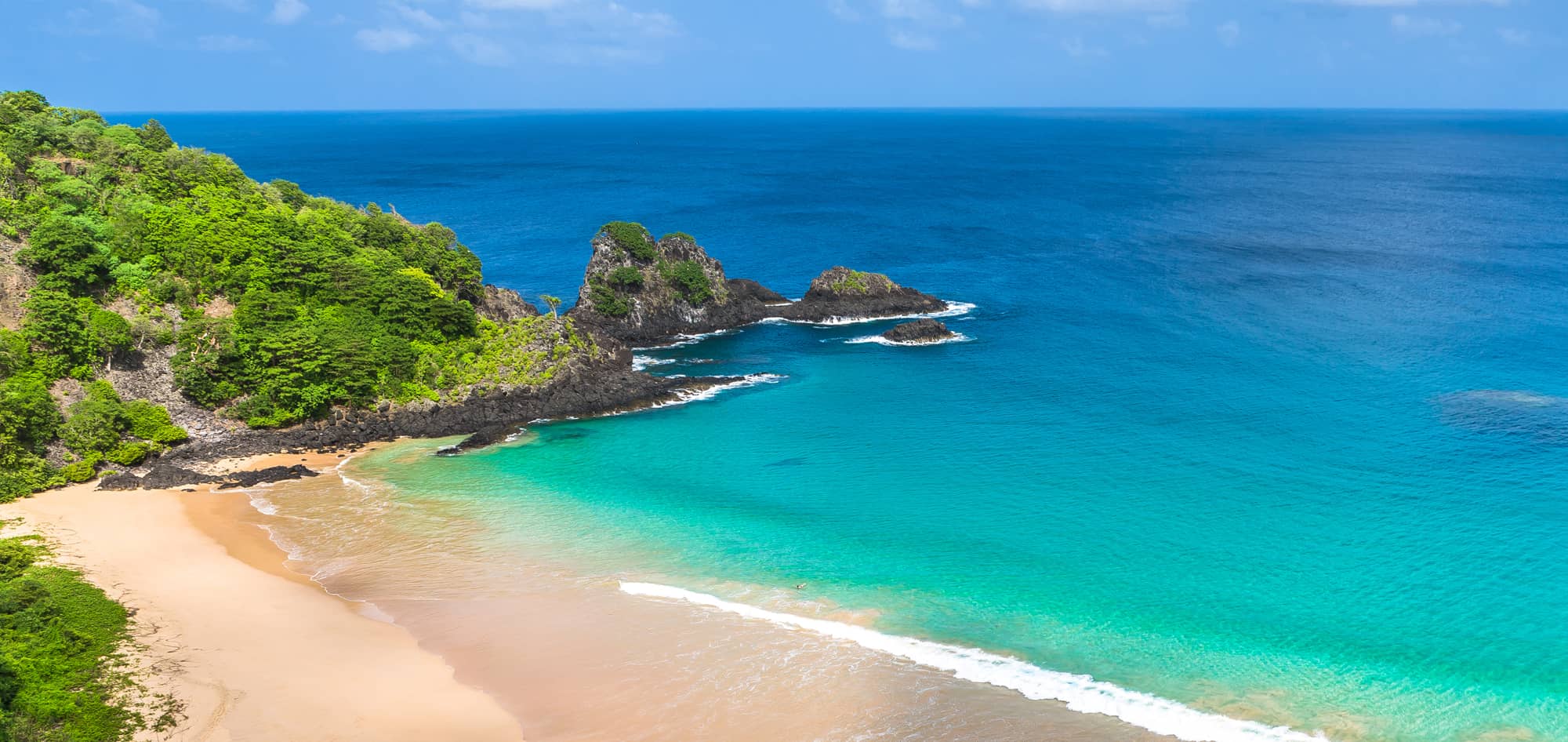This detailed aerial photograph captures a serene beach scene with crystal-clear, tropical green waters that allow the sea floor to be visible many feet past the coastline. The beach is covered in bright, tan sand, which stretches out undisturbed in the foreground. The water is relatively calm, marked only by gentle waves rolling onto the shore and crashing against several rocky outcroppings. To the left side of the image, a hillside adorned with windswept green shrubs, bushes, and trees rises up, meeting the sea where the land forms small protruding islands. As the hillside juts into the water, further rocky outcroppings coated with moss add to the picturesque landscape. The horizon sits in the upper portion of the image, where a clear sky dotted with wispy clouds meets the deep blue expanse of the ocean. The overall composition gracefully balances the greens of the vegetation, the blues of the water, and the light browns of the sand, creating a harmonious and inviting coastal vista.